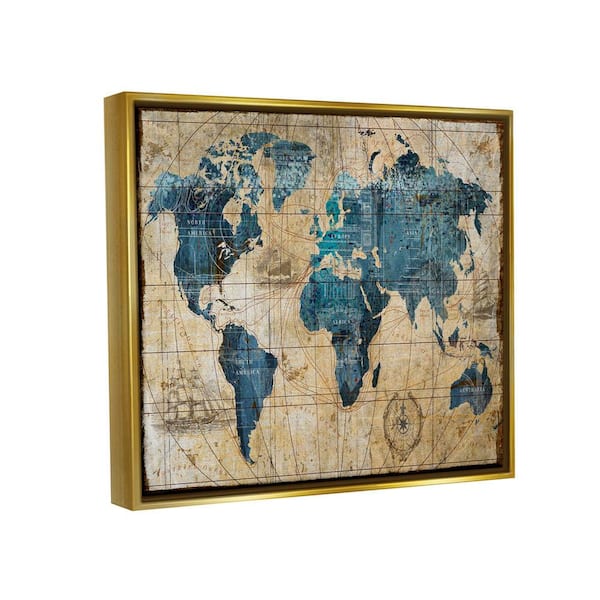This detailed photograph captures an antique-styled world map encased in a thick, golden shadow box frame. The frame surrounds an off-white, cream-colored map meticulously illustrated with various tan iterations that bring out its antique vibes. All the continents are prominently displayed, including North America, South America, Europe, Africa, Asia, Australia, and New Zealand. However, Antarctica is noticeably absent. The landmasses are rendered in dark green and shades of blue, with nuanced textures to highlight mountain ranges and landscapes. A compass, delicately drawn in pencil, is positioned at the bottom right corner, adding a navigational touch. To the bottom left, a detailed drawing of a ship, reminiscent of historical sailboats, is subtly overlaid in the background. Additionally, the map features intricate latitude and longitude lines, encapsulating the meticulous details one would expect in a classic world map.